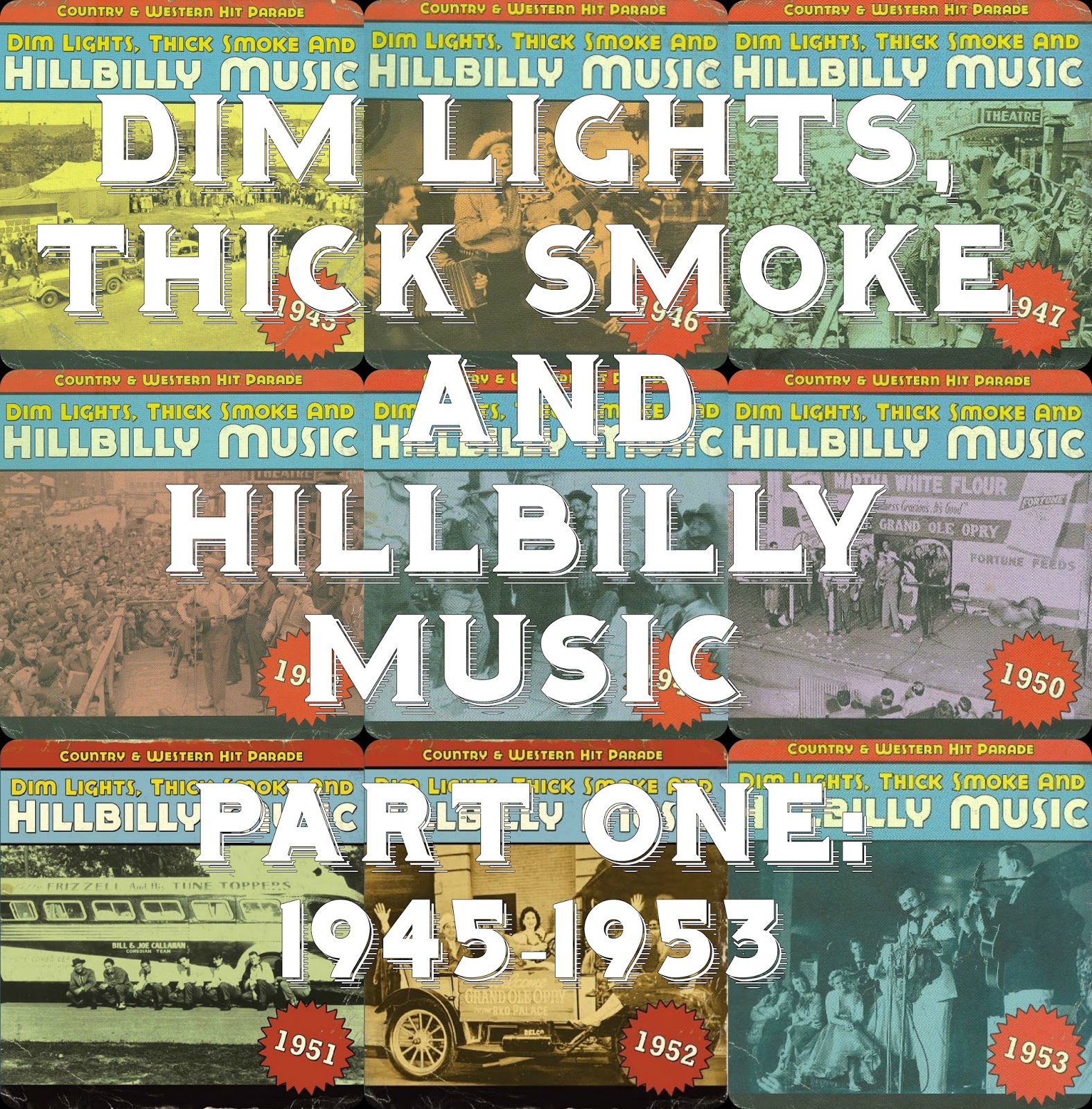The image is a square-shaped album cover, approximately 6 inches by 6 inches, featuring a collage of nine smaller album covers arranged in three rows of three. Each smaller album cover has a thin red horizontal banner at the top with yellow print reading "Country and Western Hit Parade." Below this red banner is a blue section with yellow text that says "Dim Lights, Thick Smoke," and in bold white print, it says "Hillbilly Music." Each smaller album cover also includes a black-and-white photograph, some with green or purple tints, depicting various scenes of people singing or performing. In the bottom right corner of each smaller cover, there's a red circle displaying a year, starting from 1945 in the top left and progressing to 1953 in the bottom right. Overlaying the entire collage, in bold white text, the main album cover reads "Dim Lights, Thick Smoke, and Hillbilly Music Part 1, 1945-1953."